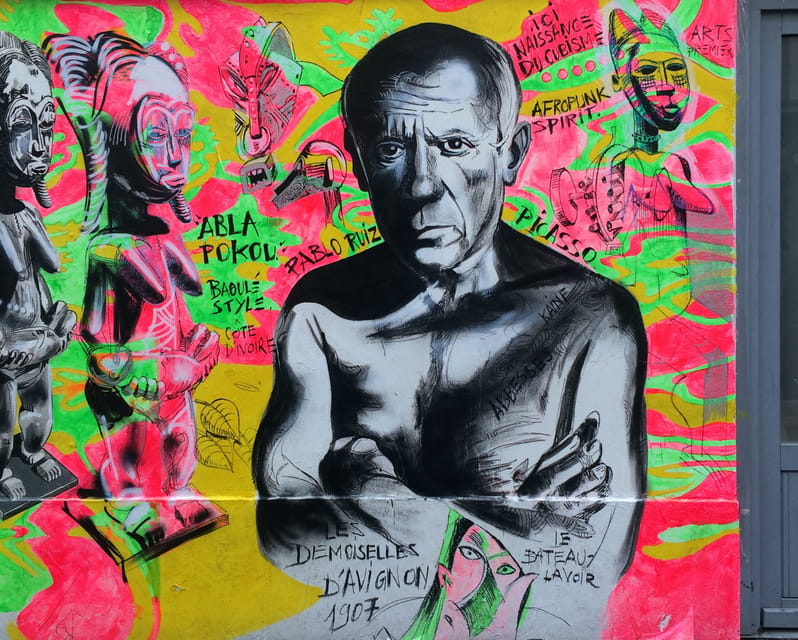The photograph, which is rectangular with longer top and bottom sides, captures an intricate piece of graffiti art on the side of a building. Dominating the frame is a black and white depiction of a shirtless man, visible from the waist up, with his arms folded across his chest and a solemn expression directed at the viewer. His bald head, adorned with sparse hair on the sides and back, adds to his distinctive, serious look. Surrounding him, the wall bursts with an array of vivid neon colors—pink, green, and yellow—that create a striking contrast to the monochromatic central figure. The background features various textures and shapes, along with artistic depictions reminiscent of African idols and structures, rendered in both black and white and color. There are also multiple texts in black, including the phrases "Afro-punk spirit Picasso," adding layers of cultural and artistic references to the scene. On the right side of the graffiti, a blue-framed single-pane window with a windowsill adds another architectural element to the vibrant tableau.